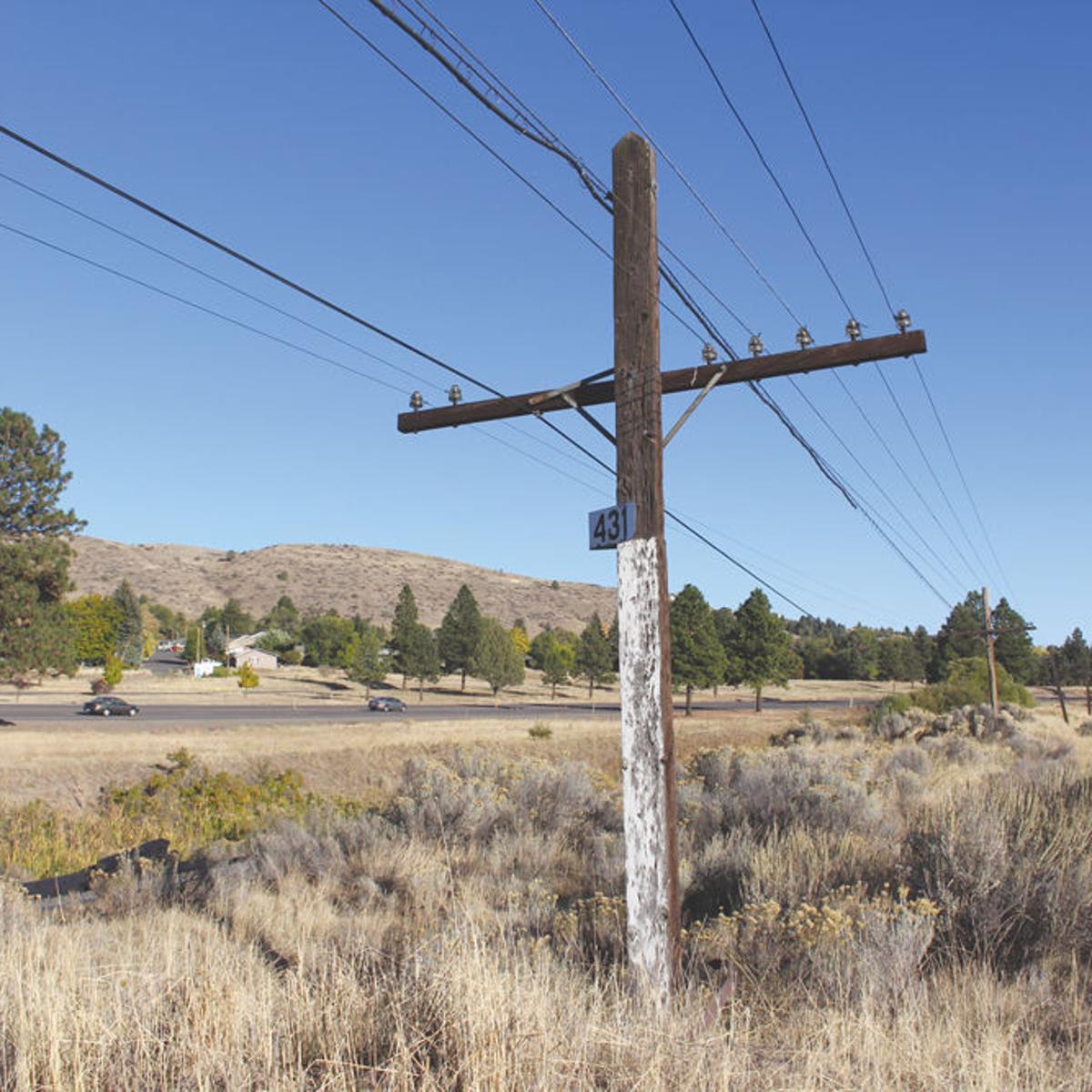This square outdoor photograph captures a rustic, rural setting dominated by a wooden power pole marked with the number "431." Situated centrally in the frame, the pole features a crossbar with glass insulators supporting the power lines. The landscape is characterized by tall, dead grasses interspersed with sporadic shrubs and patches of green brush, suggesting a dry season. To the left, a small paved two-lane road runs parallel to the power lines, where a couple of gray cars are visible driving and a few houses stand in the distance. The scene includes several green trees and a small hill in the background, all under a clear, vibrant blue sky without a single cloud, adding a sense of openness to the wide, grassy field. The image conveys a timeless, slightly dreary atmosphere, with the wooden pole and its surroundings evoking a sense of history and untouched nature.